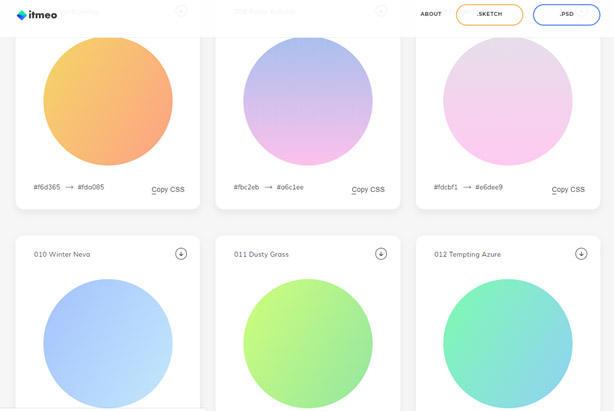In the top left corner of the image, there is a blue diamond icon accompanied by the text "ITMEO" in black. Below this, the image is divided into two rows, each containing several white squares with colored circles and text descriptions inside.

On the first row:
- The first white square contains an orange circle with the label "copy CSS" in the lower right corner.
- Next to it, there is another white square with a circle that transitions from purple at the top to pink at the bottom, also labeled "copy CSS."
- The final white square on this row houses a light pink circle, again labeled "copy CSS."

Above the set of squares on the first row, inside an orange circle, appears the text "SK Tech," which is enclosed within a blue outline that forms a stylized "PSD."

On the bottom row:
- The first white square contains a blue circle with the text "010 Winter News" above it.
- To the right, there is another white square featuring a lime green circle labeled "Dusty Grass."
- The last white square on this row contains a circle with a gradient mix of blue and green, identified as "012 Tempting Azure."